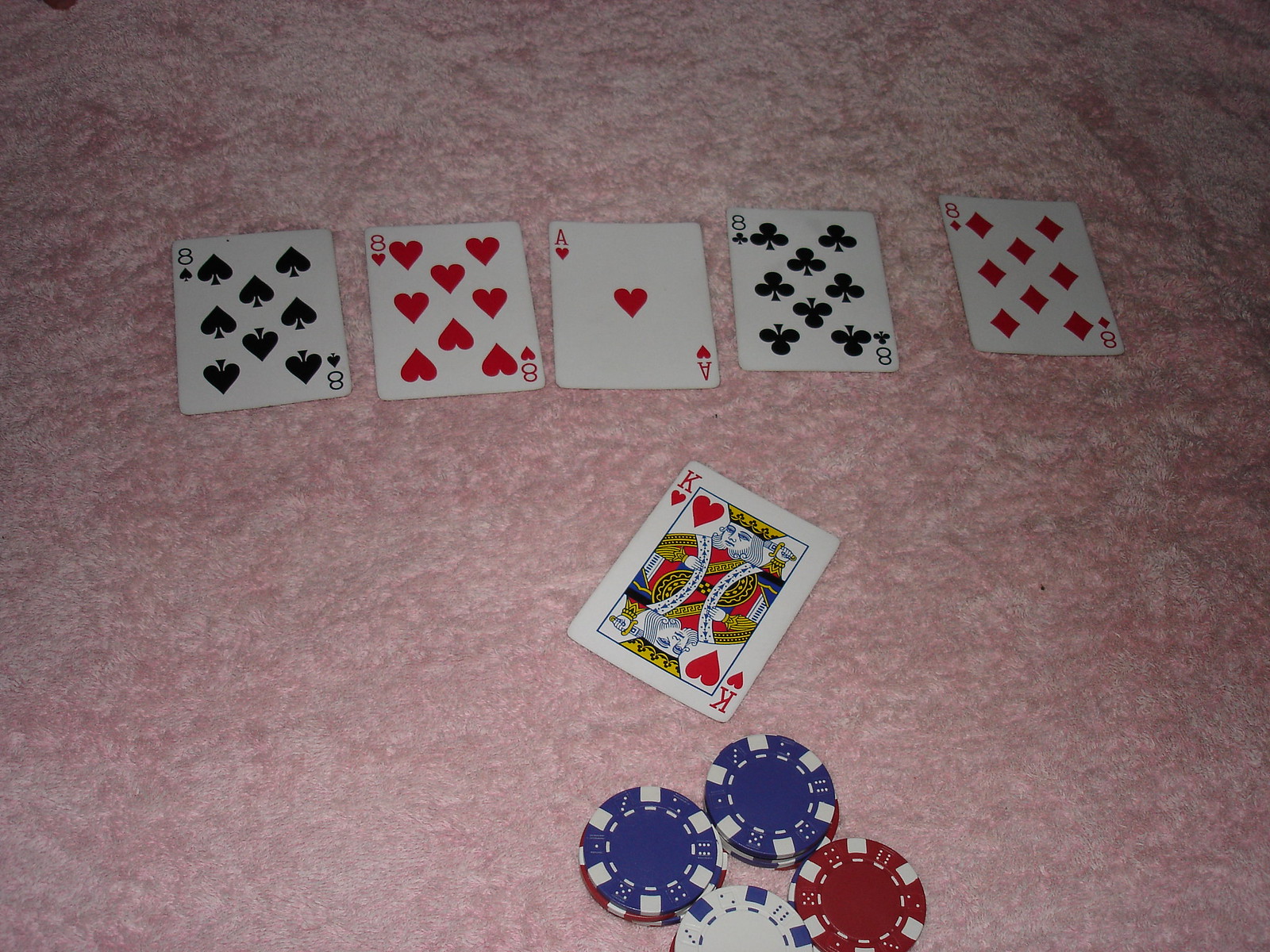The image displays a set of playing cards meticulously arranged on a rough-textured pale pink surface. Centered in the image, five cards are laid out in a straight horizontal row. From left to right, the cards are as follows: Eight of Spades, Eight of Hearts, Ace of Spades, Eight of Clubs, and Eight of Diamonds. Directly below this row, a King of Hearts card is positioned at a slight diagonal angle. Beneath the King of Hearts, a collection of gambling chips is neatly organized in a square formation. These chips are in three distinct colors: blue, red, and white, adding a touch of vibrancy to the scene.